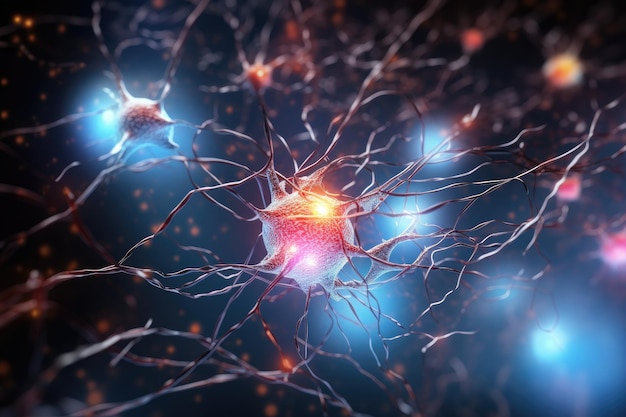The image is a horizontally aligned rectangular digital creation, roughly four inches wide and three inches high. It features an artistic representation of synapses or neural connections. The background is predominantly solid black, accentuating the intricate foreground. The main focus is a large, circular hub at the center, emitting a yellow and white light with an orangish and cream-colored zig-zag pattern. Grayish fibers with white tips radiate from this central hub in all directions, connecting to smaller, round objects throughout the image. These objects have blue halos and white centers and are partially blurred in the background, creating depth. Additional scattered lights in hues of yellow, blue, and pink add to the intricate web of connections, evoking the idea of a complex, interconnected neural network. The overall effect is a vivid and detailed visualization of what could be a nervous system or cellular synapses, with vibrant colors and glowing lights highlighting the connectivity.